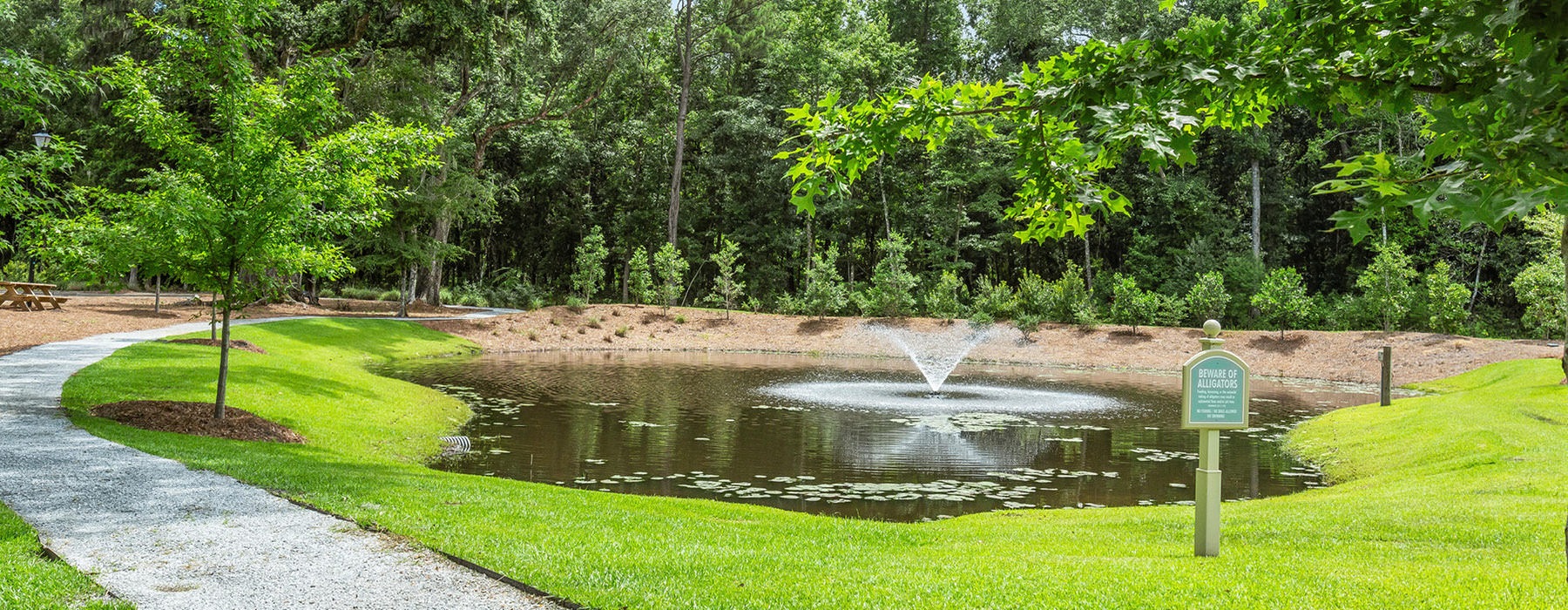This is a realistic photograph, taken during daylight, capturing a serene park scene with excellent lighting. The composition features a long, horizontal rectangle format. In the foreground, a manicured, plush green lawn stretches from the left to the middle, encircling a small pond situated in the center of the image. The pond, adorned with lily pads, has a small fountain that elegantly sprays water in an upside-down triangle formation.

On the left side, a white gravel stone path curves in a 'C' shape, accompanied by a freshly planted small tree and a mulched area hosting a wooden picnic table. Further back, the landscape transitions into an edge of a dense forest, with a variety of lush, deep green trees and bushes creating a tranquil backdrop. There is also a mulched area with benches that appear to be positioned on tan-colored mulch. Also, a sign with a green background and white text - possibly about local wildlife - is visible, though the inscription is unclear. Overall, the scene exudes calmness and natural beauty, making it a perfect setting for relaxation.